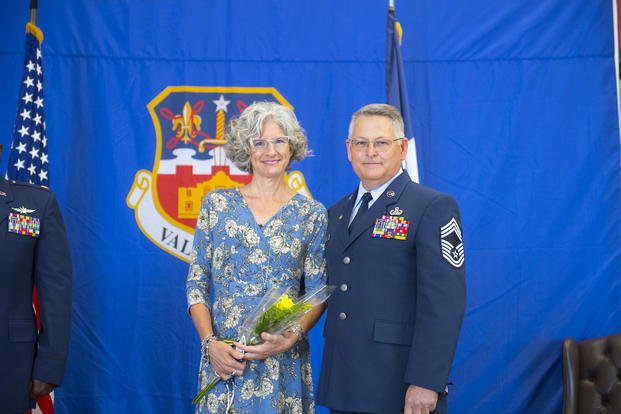This indoor photograph captures a ceremonial moment featuring two prominently positioned individuals, presumably a couple, based on their closeness and attire indicative of a formal event. The woman on the left is wearing a blue dress adorned with white floral patterns, her gray, wavy hair styled above shoulder length, and she's holding a small bouquet of yellow flowers. She is smiling, adding warmth to the scene. Standing to her right is a man with short gray hair and glasses, dressed in a navy blue military uniform embellished with medals and patches that signify his distinguished service, emphasizing his military background. Both individuals are Caucasian, evident from their fair skin. They are positioned against a blue backdrop featuring a central logo. Partially visible on the left is another individual in a similar military uniform, though only their arm and shoulder are seen alongside a USA flag, hinting at a patriotic or official setting. The bottom right corner reveals a black sofa, adding a touch of the indoor environment.